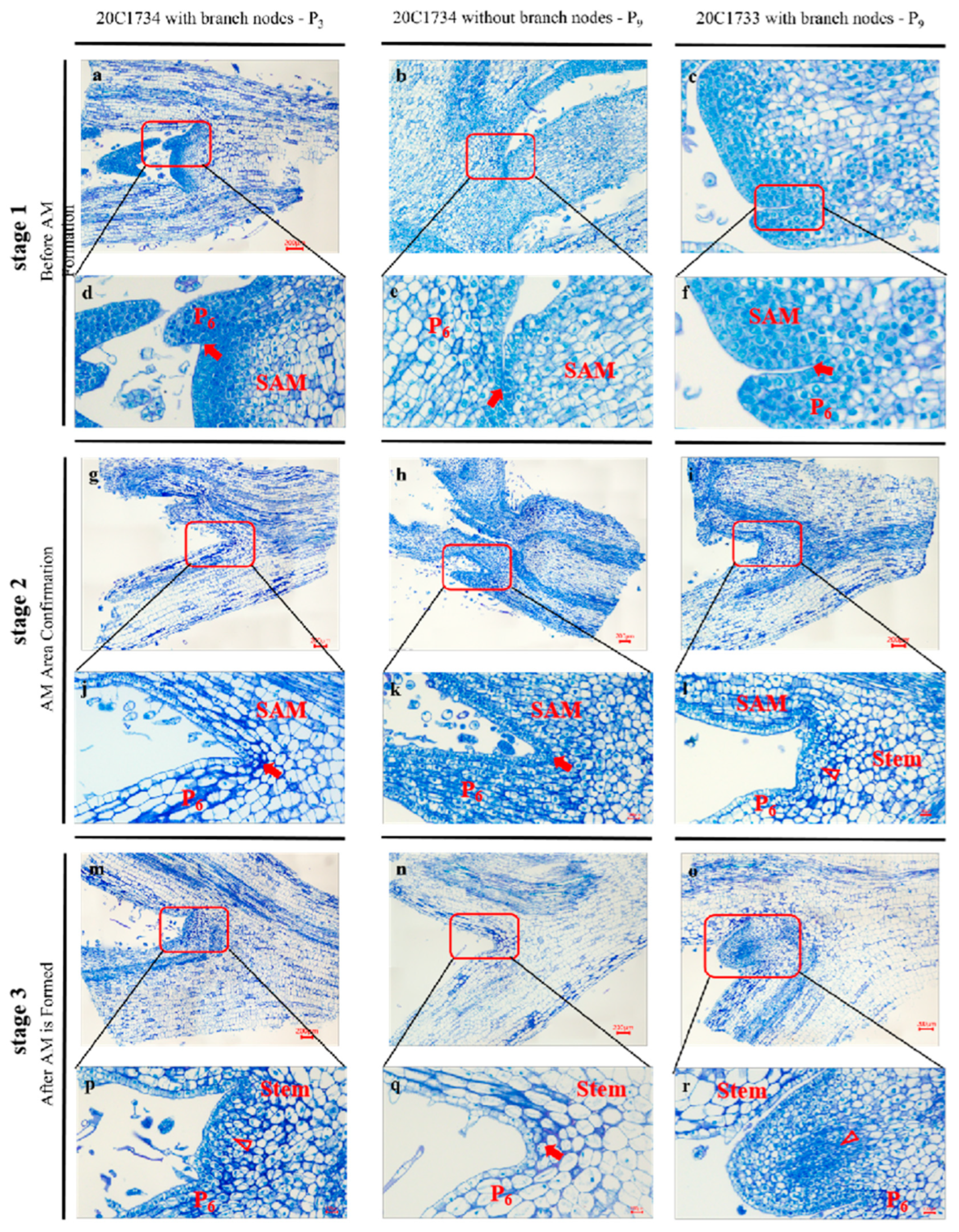The image is a detailed 18-panel diagram displayed on a white background in a vertical rectangle format, with six rows and three columns of uniformly sized panels. Each panel features microscopic scans that depict blue-colored molecules, with annotations in black text, red rectangles, and arrows highlighting key areas. The panels are organized into three stages of a process: 

1. **Stage 1: Before A.M.**
   - Panels are labeled with identifiers such as "M203 C1734 with branch nodes P220 C1734" and "without branch nodes P920 C1733." 

2. **Stage 2: A.M. Area Confirmation**
   - Includes additional annotations like "Sam, Sam, Sam" and "Stem."

3. **Stage 3: After A.M. is Formed**
   - Each panel continues to feature intricate blue and white microscopic imagery with red rectangles marking significant details. 

Black titles at the top of each column correspond to narrow horizontal bars, though the text is too small to read. Along the left side, black text tilted at a 90-degree angle titles sections of rows, indicating broader categories or descriptions shared by groups of two rows each. The light blue color is predominantly dotted throughout the imagery, emphasizing the molecular structures and the specific areas highlighted in red.